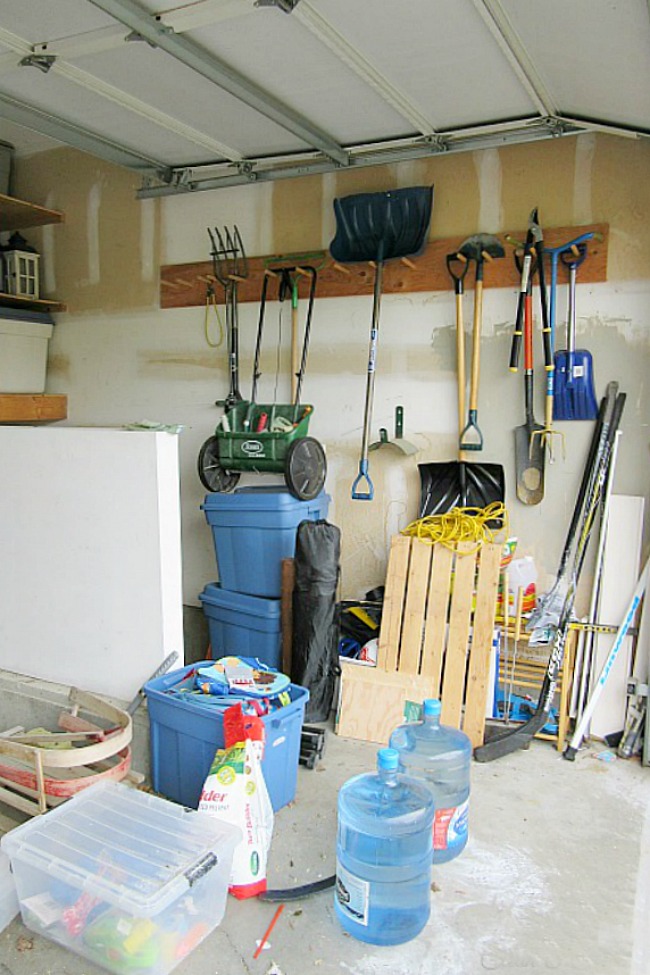This daytime photo captures a somewhat cluttered garage with the white garage door open and sunlight streaming in. Along the top part of the image, a pegboard hangs various lawn and garden tools, including a pitchfork, a fertilizer spreader, a large snow shovel, smaller snow shovels, a spade, a regular shovel, and bush trimming shears. The concrete floor beneath features several blue five-gallon storage totes, stacked and scattered, along with a smaller clear tote. Additionally, the floor hosts an assortment of items, such as a wooden snow sled, a hockey stick, a bag of fertilizer, a couple of five-gallon water bottles, and possibly a chair stored in a bag. The scene is completed by stacks of wood and what appears to be a coil of yellow rope, giving the garage an organized yet busy appearance.